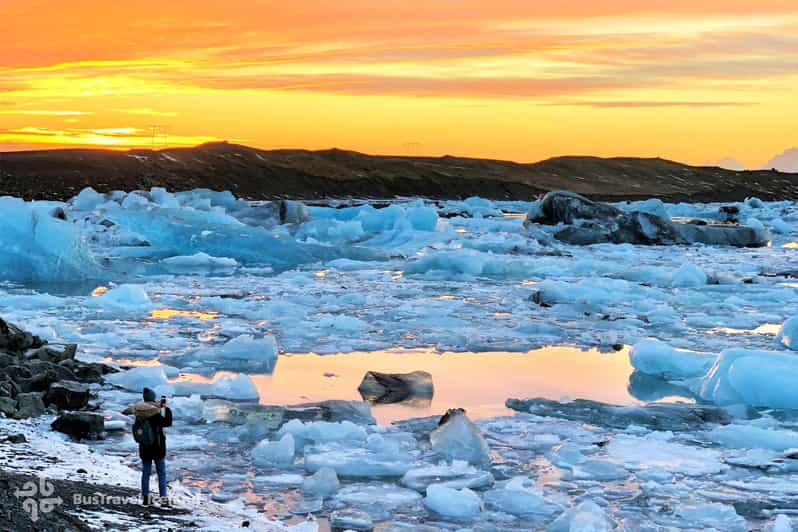In this stunning image, we are looking at a vast, frozen coastal area, possibly located in Greenland or the Arctic. The scene is dominated by an expansive, slushy sea of broken ice chunks in varying shades of light blue and white, interspersed with small patches of open water. In the foreground, on the bottom left corner, stands a woman dressed warmly in a black jacket with brown fur edging on the hood, blue jeans, a black backpack, and a knit hat, clearly prepared for the cold. She holds a phone, possibly capturing the breathtaking scenery in front of her while standing on a stretch of black and gray gravel. Beyond the icy expanse in the foreground, we see a backdrop of black gravel or rocky terrain that transitions into rolling brown hills and distant mountainous ranges. The sky is ablaze with the hues of a vibrant sunset—vivid oranges, reds, maroons, yellows, and purples blending together, with scattered clouds adding texture to the scene. This mesmerizing view captures the serene yet dynamic beauty of nature at twilight.